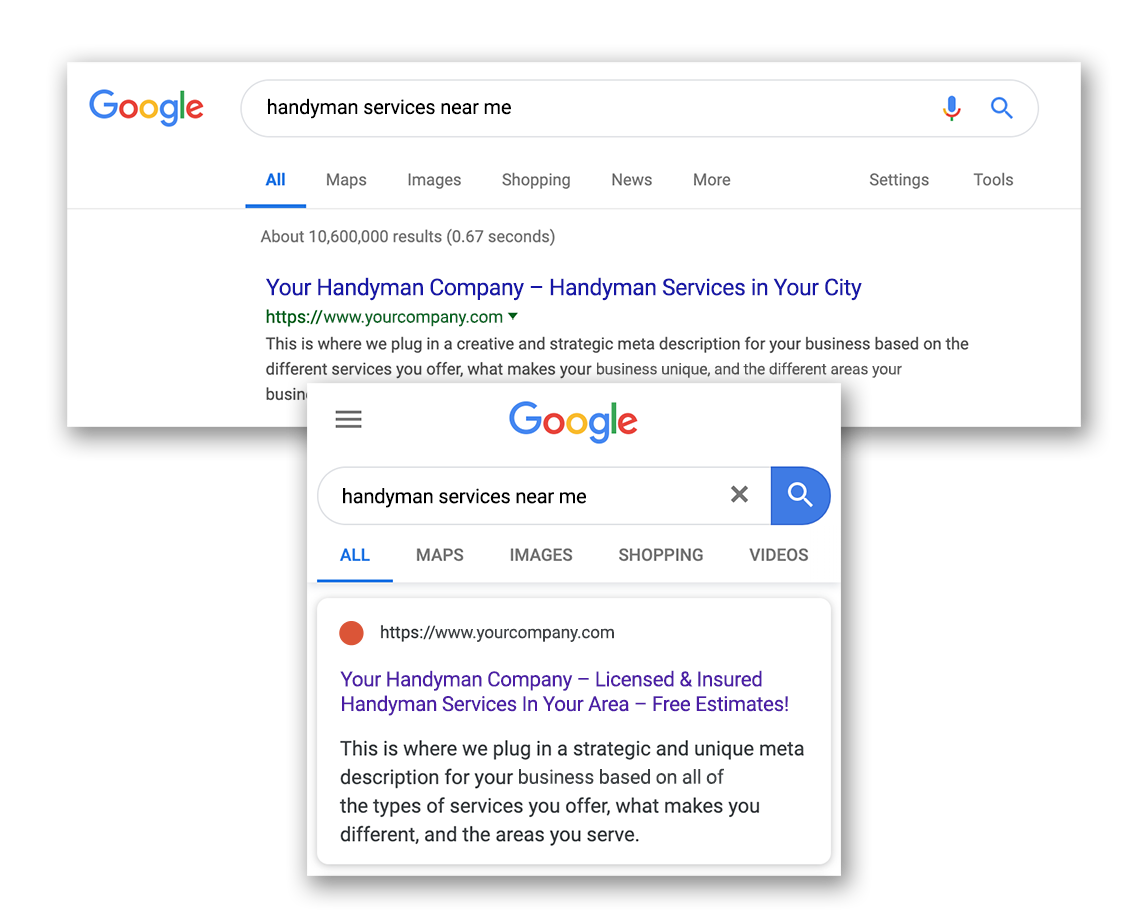The image depicts a Google search results page. On the left side of the page, the Google logo is prominently displayed. Below it, there's an oval-shaped search bar with the query "handyman services near me" typed out in black text. To the right side of this search bar, there's a blue pill-shaped microphone icon positioned on a red stand, and a dark blue magnifying glass symbol.

Below the search bar, a series of tabs can be seen: "All," "Maps," "Images," "Shopping," "News," and "More." The "All" tab is currently selected, evident from the text being blue and underlined in the same color. To the far right of these tabs, the options "Settings" and "Tools" are listed.

The first search result is a hyperlink in blue text, reading "Your Handyman Company - Handyman Services in Your City." Beneath this, the URL "http://www.yourcompany.com" is displayed in green with a downward arrow next to it.

The second search result, displayed in a separate rectangle, shows a similar format: "Your Handyman Company, Licensed and Insured, Handyman Services, In Your Area, Free Estimates" in blue hyperlinked text, which has turned purple, indicating that it has been clicked. Below this, in black text, is a placeholder description stating, "This is where we plug in a strategic and unique meta description for your business based on all of the types of services you offer, what makes you different, and the area you serve."